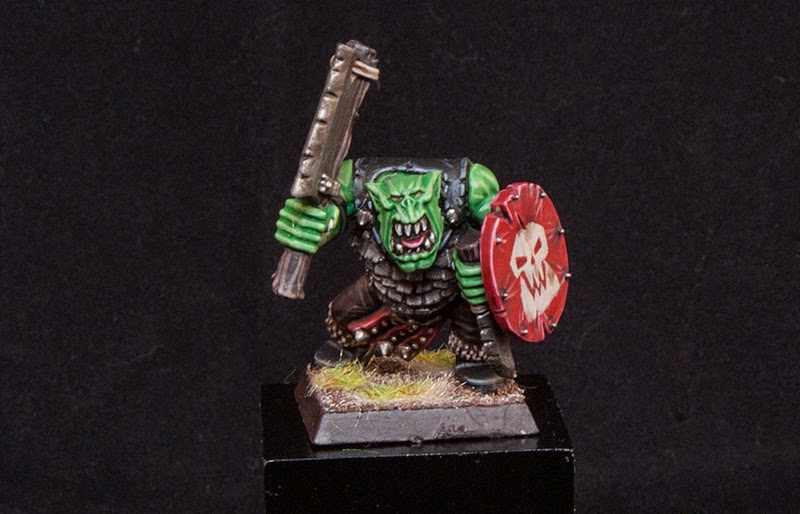This image showcases a highly detailed figurine of a green goblin-like creature, prominently positioned against a solid black background. The figurine stands on a square base adorned with patches of grass, which rests atop a small wooden block. The goblin is equipped with imposing warrior-style attire, featuring dark, sleeveless metal plate armor, leather pants, and boots. Additional details include spiked circular accessories around its ankles and a small spiked skirt.

The creature has distinct, pointed green ears and an open mouth, revealing sharp white teeth and a visible pink tongue. In its right hand, it wields a crudely fashioned weapon, resembling a wooden bat with a metal blade fastened with nicks and ties, suggesting a brutal, makeshift design. Its left hand holds a large, red leather shield, notable for its white orc skull emblem and visible rivets that hold the stretched material in place. The figurine appears to be slightly crouched or bending its knees, adding a dynamic, lifelike quality to its stance.